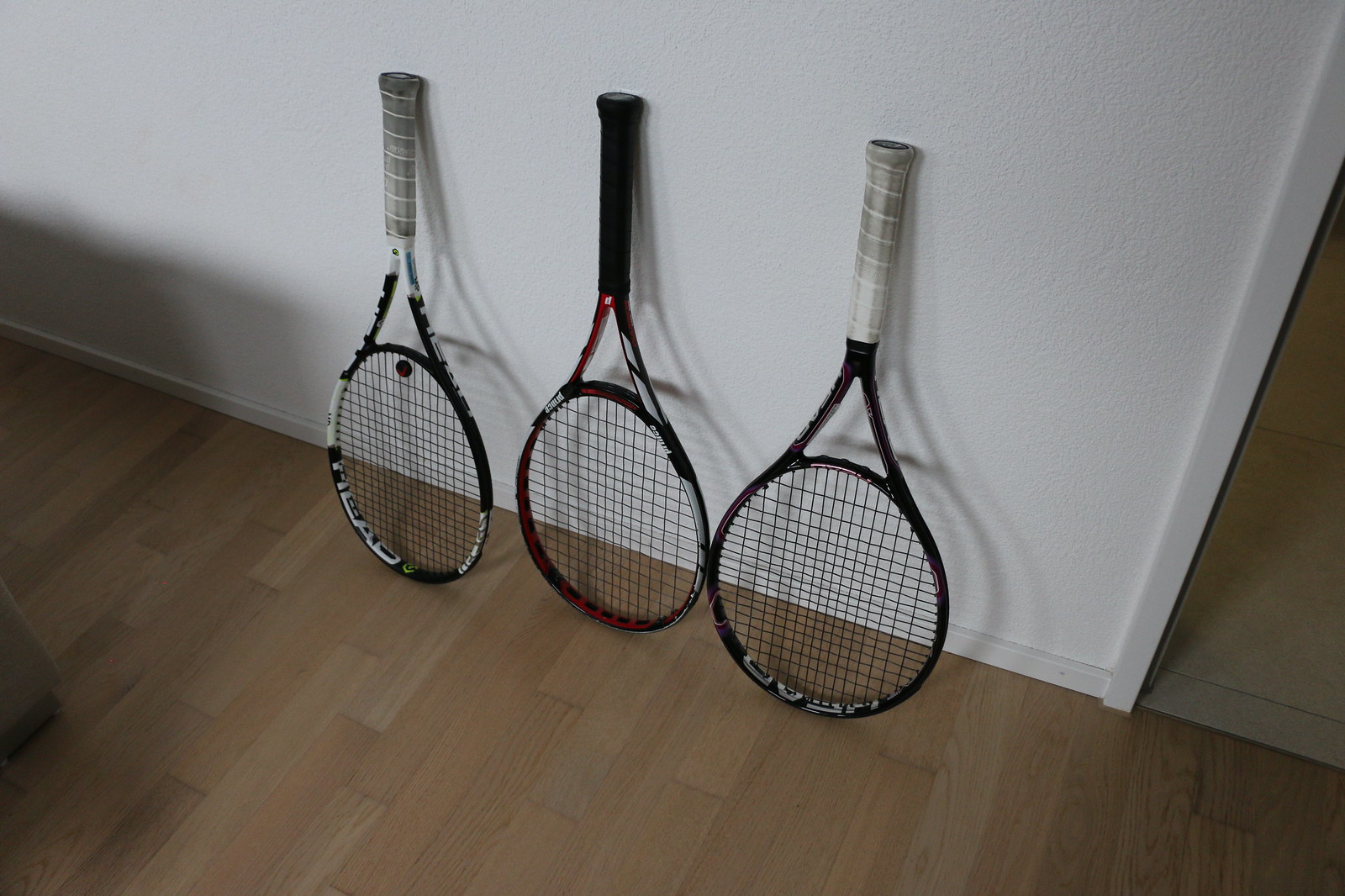This photograph depicts an indoor setting, likely a home, featuring a distinctive arrangement of three tennis rackets leaning upside down against a white wall, which has white baseboards. The light wood floor, possibly laminated, contrasts with the white wall and baseboards. To the right, an open doorway reveals a tiled floor leading into another room.

The tennis rackets are neatly lined up in a row with their handles propped against the wall and their string areas touching the floor. The racket on the left has a notably dirty grip, once white but now a dark grey, and a black and white design, suggesting it is a Head brand. The middle racket features a black handle with a predominantly black and white design, accented with red. The racket on the right has a similar dirty and greyed handle, originally wrapped in white, and shares the black and white design of the Head brand. All three rackets are precisely positioned, offering a balanced and orderly focal point against the minimalist backdrop of the white wall and light wooden floor.